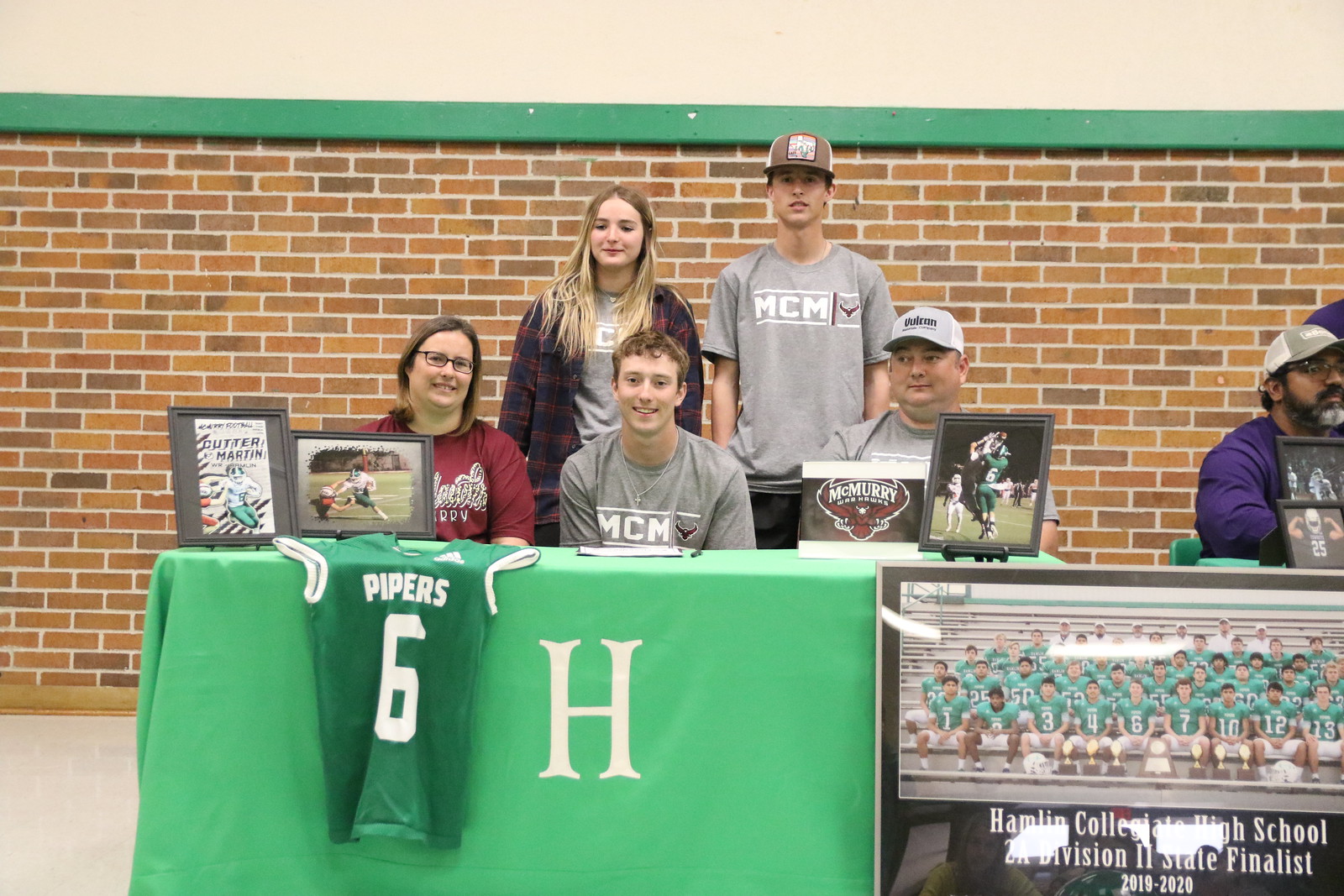The photograph captures a group of five teenagers, predominantly Caucasian, seated and standing around a table draped with a light green tablecloth bearing a prominent white capital letter "H" at the front. The table displays a green basketball jersey with the name "Pipers" and the number "6" in white, alongside several framed photographs showcasing football highlights in gray frames. A standout photograph on the bottom right features a team from Hamilton Collegiate High School, labeled "2nd Division, 2nd State Finalists 2019 to 2020," showing about 30 players in light green jerseys seated in bleachers.

In the image, three individuals are sitting—one girl and two boys—while two others stand behind them. Seated on the left is a girl with long brunette hair and glasses, wearing a dark red T-shirt. Beside her is a boy with short curly hair, dressed in a gray MCM T-shirt featuring a hawk logo, who looks directly at the camera. The boy on the right, also in a gray MCM T-shirt, wears a gray and white baseball hat and looks off to the left.

Standing behind them, a teenage girl with blonde hair reaching past her shoulders dons the same gray MCM T-shirt and a red and blue plaid jacket, looking downward. Next to her, another teenage boy in a gray MCM T-shirt and a mainly brown hat is partially visible. The backdrop transitions from a light orange brick wall to a plain cream-colored wall with a green stripe running horizontally. To the far right, partially cropped out, is an unrelated individual in a purple shirt, sporting a black beard, glasses, and a gray and white hat.